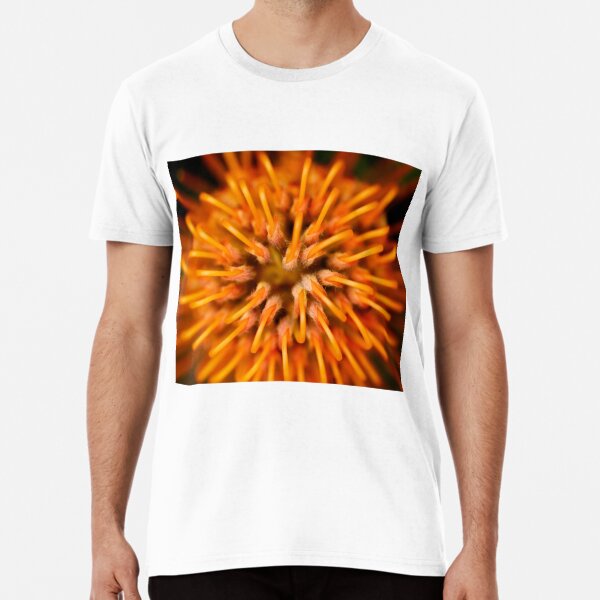The image features a Caucasian male wearing a white t-shirt adorned with a bold, square graphic in the center. The graphic, occupying the chest and upper stomach area, is a bright and intricate design that appears to be a close-up of an orange and yellow flower or possibly a creature from a coral reef, characterized by pointy, spiky elements with a dark background. The image is cropped just below his chin, revealing his somewhat hairy arms relaxed by his sides and faint facial hair growing on his neck. He wears black shorts without any visible logos. Set against a plain white, off-white background, the focus is clearly on the t-shirt design, suggesting it might be an example of apparel being showcased for online sale.